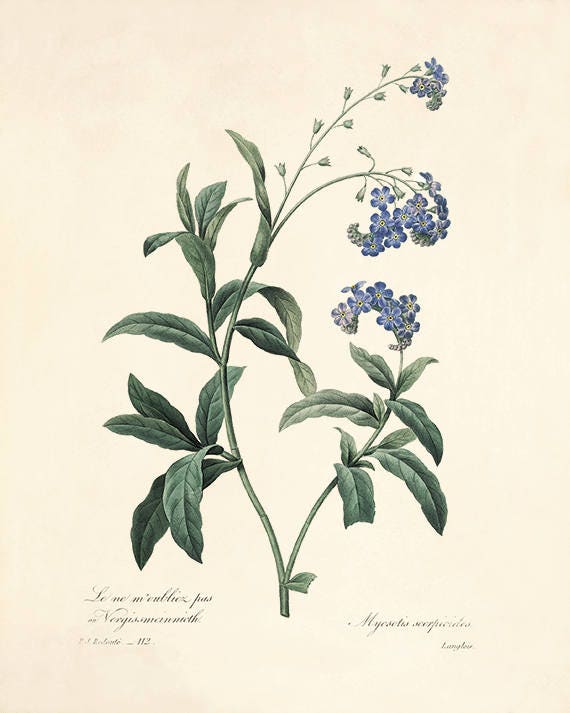This detailed drawing of a plant is set against an elegant, light beige background, reminiscent of old parchment. The image is approximately five inches high and four inches wide, creating a rectangular shape. Starting from the bottom center, a singular green stalk emerges and quickly splits into a V-formation, creating two main branches. The left branch initially bows out towards the left before arching back to the right, nearly reaching the top of the illustration. The right branch points upward and extends about halfway up the page. Both branches feature dark green, elliptical-shaped leaves that grow in smaller clusters as they ascend. At the very ends of the branches, small clusters of bluish-purple flowers with yellow centers bloom, with some buds yet to open. The background subtly transitions to a hint of pink near the top and bottom left corners. Additionally, there is cursive script at the bottom left and right corners, appearing to be in French, though it is too small to decipher clearly.